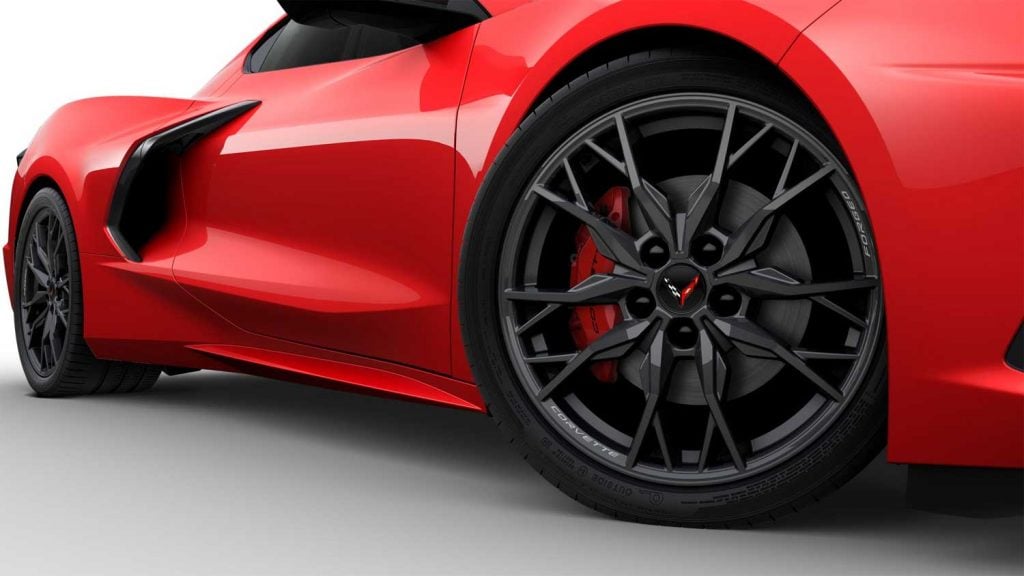The photograph features a striking cherry red sports car, prominently occupying most of the image with emphasis on its front section and wheels. The shot is angled from the ground looking up, capturing the dynamic presence of the car. Only the front half of the vehicle is visible, with the rear and rest of the sports car cut off from view. The sleek car's polished and well-maintained appearance suggests it's primed for performance.

Intricate details of the black tires are highlighted, showcasing black rims with a unique Y-shaped emblem at the center—one arm of the Y resembles a checkered flag, while the other resembles a red ribbon, tying into the car's overall red theme. The tires are slim and complemented by the black frame that subtly accents the vehicle. The door area features a distinctive black accent, and the car's futuristic design is further emphasized by the sculpted black side mirrors and window outlines. The entire scene underscores the sports car's elegance and speed, making it an irresistible purchase for enthusiasts.